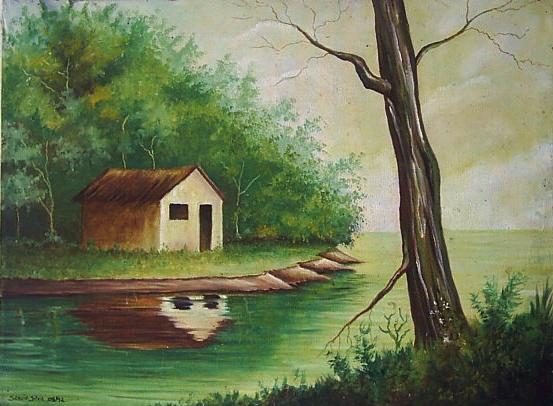This painting depicts a serene countryside scene with a small, quaint house situated on a grassy plot of land that slopes down to a vibrant green lake. The house, positioned to the left, features a yellowish-whitish façade with a slightly rusted brown tin roof, and dark brown door and window cutouts. Behind the house, a cluster of green trees adds depth to the background. The sky has a cloudy, yellowish, and greenish hue, contributing to the calm yet slightly eerie atmosphere. In the foreground, on a grassy knoll at the edge of the lake, stands a wiry, leafless tree with thin, outstretched branches. The green-colored water of the lake reflects the house, mirroring its image below. Various shades of green, brown, yellow, and off-white dominate the scene, creating a harmoniously rustic palette.